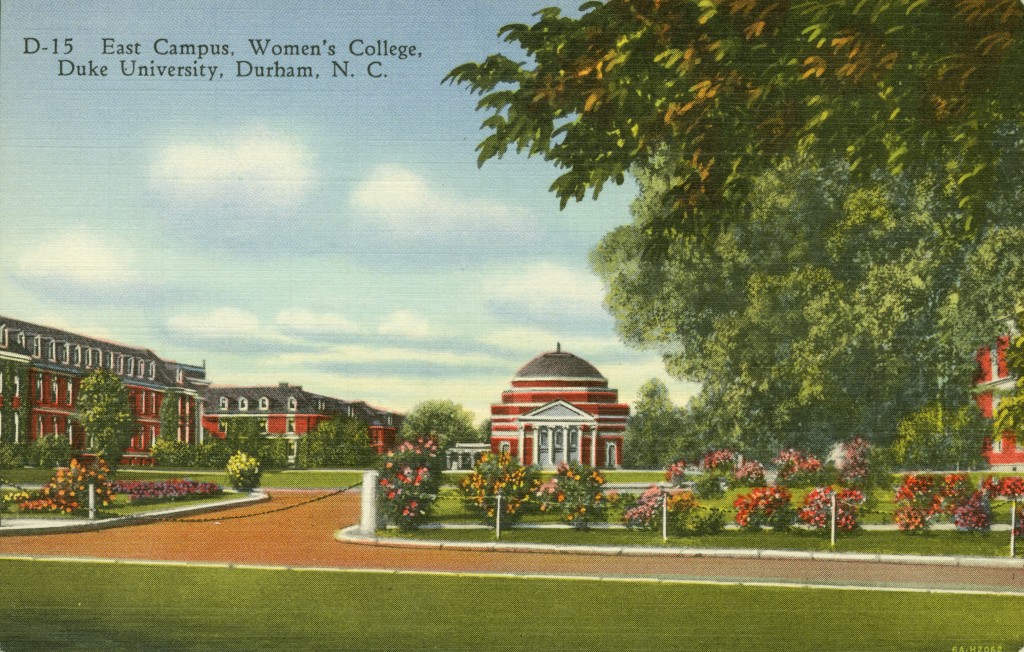This image, styled as a painting or drawing, prominently features the East Campus Women's College at Duke University, Durham, North Carolina. The scene is likely from the front of a postcard and includes the label "D15 East Campus Women's College, Duke University, Durham, NC" in the upper left corner. The picturesque campus showcases a blend of rich details: large, vibrant trees occupy the upper right, offsetting a meticulously manicured lawn interspersed with multicolored flower beds. 

A red brick walkway, possibly a sidewalk, threads its way through the scene from the lower left foreground to the center, extending into the distance. This walkway is flanked by neatly trimmed lawns and abundant flower patches. Mid-background left are red-brick buildings with black roofs, adding to the campus's charm. Dominating the central portion, a striking building commands attention; it is characterized by its reddish-brick construction, cylindrical white-columned facade, and possibly a conical or cylindrical roof, further enhancing the architectural aesthetics of the campus. This detailed representation captures the essence of a serene and visually appealing college environment.